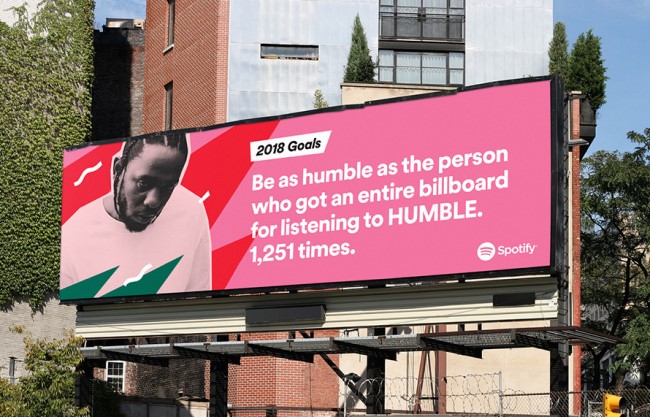This color photograph captures a large Spotify billboard set against a pink background with red and green geometric shapes. The billboard, situated on a brown wooden pole in front of a brick building, features a photograph of an African-American man, likely Kendrick Lamar, with dreadlocks and a white t-shirt. The billboard's top section displays a white banner with the text "2018 goals" in black font. Below that, in white font, it reads, "Be as humble as the person who got an entire billboard for listening to Humble 1,251 times." In the bottom right corner, "Spotify" and its logo are clearly visible. The setting includes a blue sky, some green trees, a gray building with vines, another brick building, and a fence at the bottom, suggesting a daytime outdoor environment.